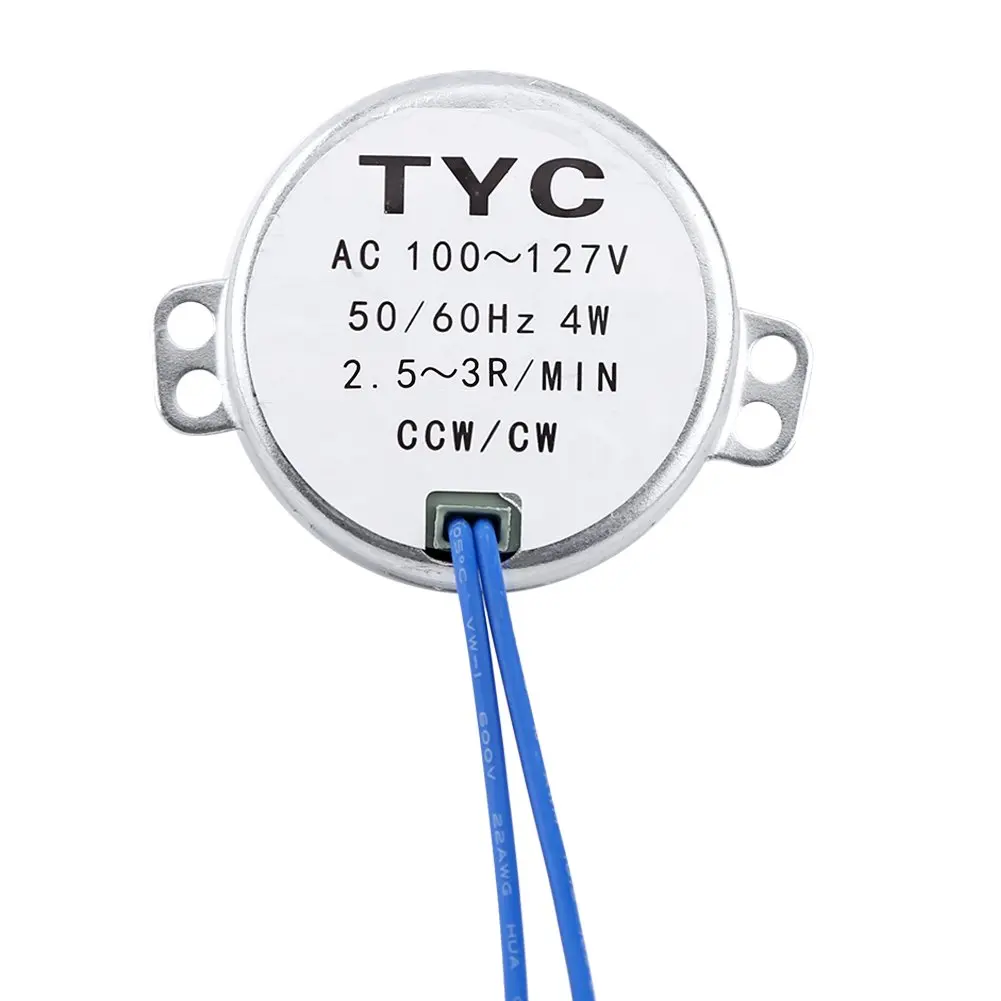The image showcases a silver, circular electrical component centered on a solid white background. Flanking the disc on each side are two protruding ears, each featuring a hole, presumably for screwing or fastening the component into place. Emerging from the bottom of the disc are two thin blue wires extending out of the frame. Affixed to the front of the silver disc is a white sticker with black text detailing its specifications: 

- **TYC** at the top in a bold font
- **AC 100 ~ 127V** on the next line
- **50/60 Hz, 4W** 
- **2.5 ~ 3R/MIN**
- **CCW/CW**

The component's structural and textual features, as well as its wiring, suggest a piece used in electrical applications, emphasizing its function and installation specifics.